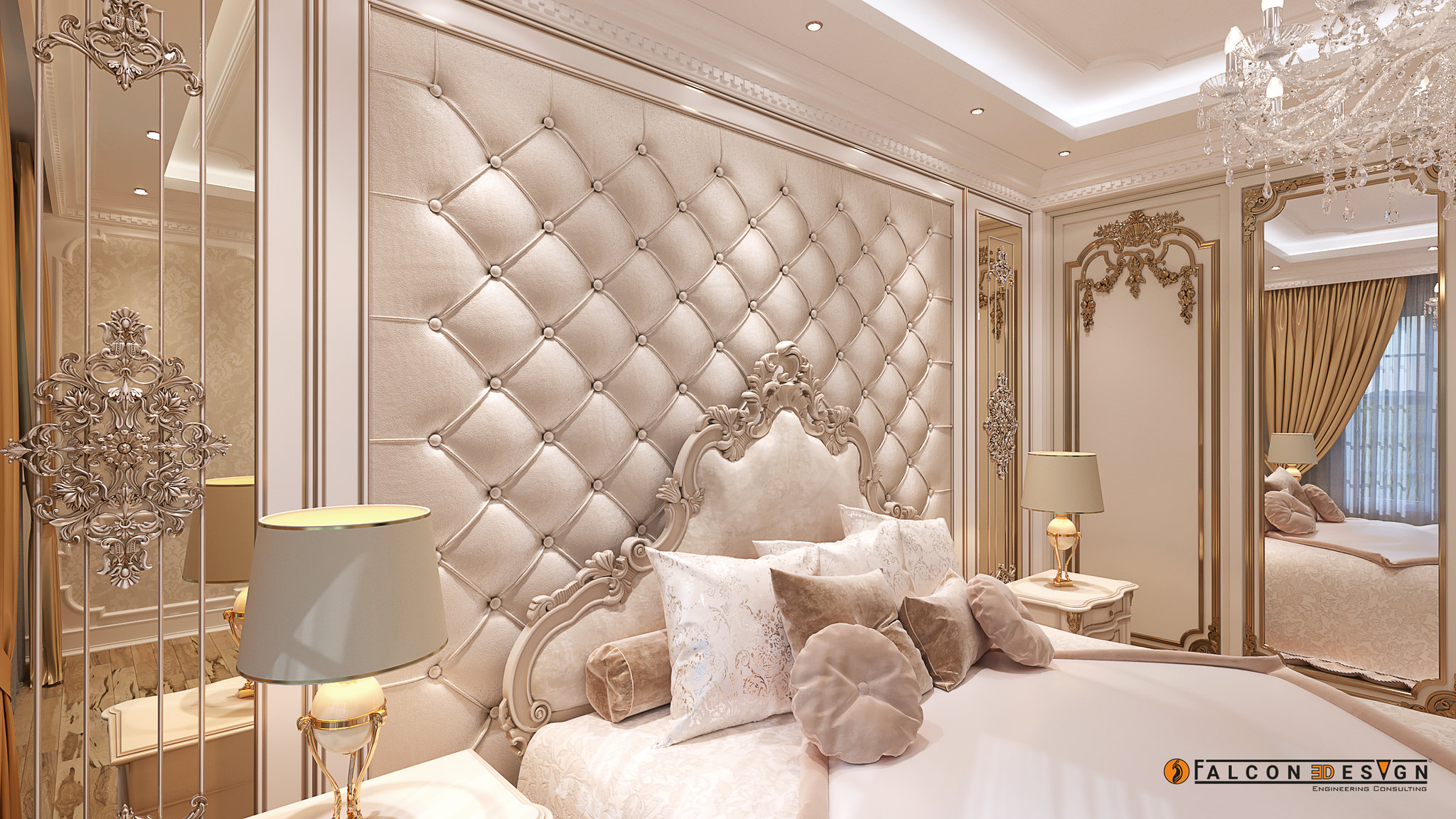The photograph captures an opulent bedroom with a light pink and champagne color scheme, designed by Falcon Design as noted in the bottom right-hand corner. The room features a luxurious fabric-covered back wall that is tufted with visible buttons, adding a cushioned, textured look. This wall seamlessly integrates with an ornate headboard, which has a wooden border and a fabric center matching the wall’s champagne tone.

The bed is adorned with a spread in a peachy-pink hue, complemented by a variety of pillows, including three pink square pillows, several decorative pillows of different shapes—round, square, and rectangular—and additional champagne-colored pillows. Each pillow arrangement enhances the bed’s lush appearance.

On the back wall to the right, a floor-to-ceiling mirror reflects the intricate details of the room, including the vaulted white ceiling studded with small circular lights, and a chandelier in the top right corner, which features delicate hanging jewels. A pair of nightstands flanks the bed, each hosting decorative gold and white table lamps with quilted patterns on the shades.

A curtain in a brownish-golden tint adds warmth to the setup, while a silver metallic design element on the left side introduces a touch of modernity to the classic decor. The overall ambiance of the bedroom is one of refined luxury, merging palatial elements with contemporary design sensibilities.